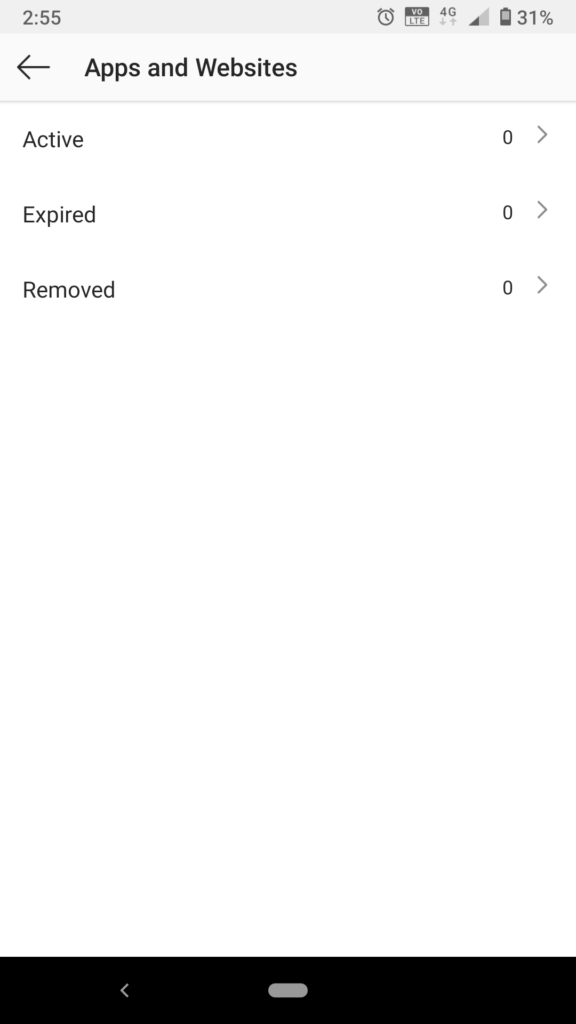This is a detailed screenshot from a mobile phone. At the very top of the screen, a small gray bar displays various pieces of information in gray font and icons. On the upper left, the time is shown as 2:55. On the right side of this bar, an array of icons appears sequentially: an alarm clock icon, a "VDLTE" label, a "4G" label indicating the mobile network type, a mobile signal strength icon displaying two out of five bars, and a battery icon indicating the battery level at 31%.

Directly below this top bar is a gray rectangle featuring a black left-pointing arrow and the text "Apps and Websites". Underneath this section, a small gray bar divides the content further.

Following this is a white section with categorized lists and corresponding arrows indicating navigation. The first category, "Active," displays a count of zero with a right-pointing arrow. Below it, the "Expired" category also shows a count of zero and a right-pointing arrow. Lastly, the "Removed" category mirrors the same layout, with a count of zero and a right-pointing arrow. 

At the very bottom of the screen, a black navigation bar is present. Centrally located within this black bar is a gray home button. To the left of the home button, there is another arrow pointing left, presumably for navigating back to the previous screen.

This detailed description encompasses all visible elements within the screenshot.